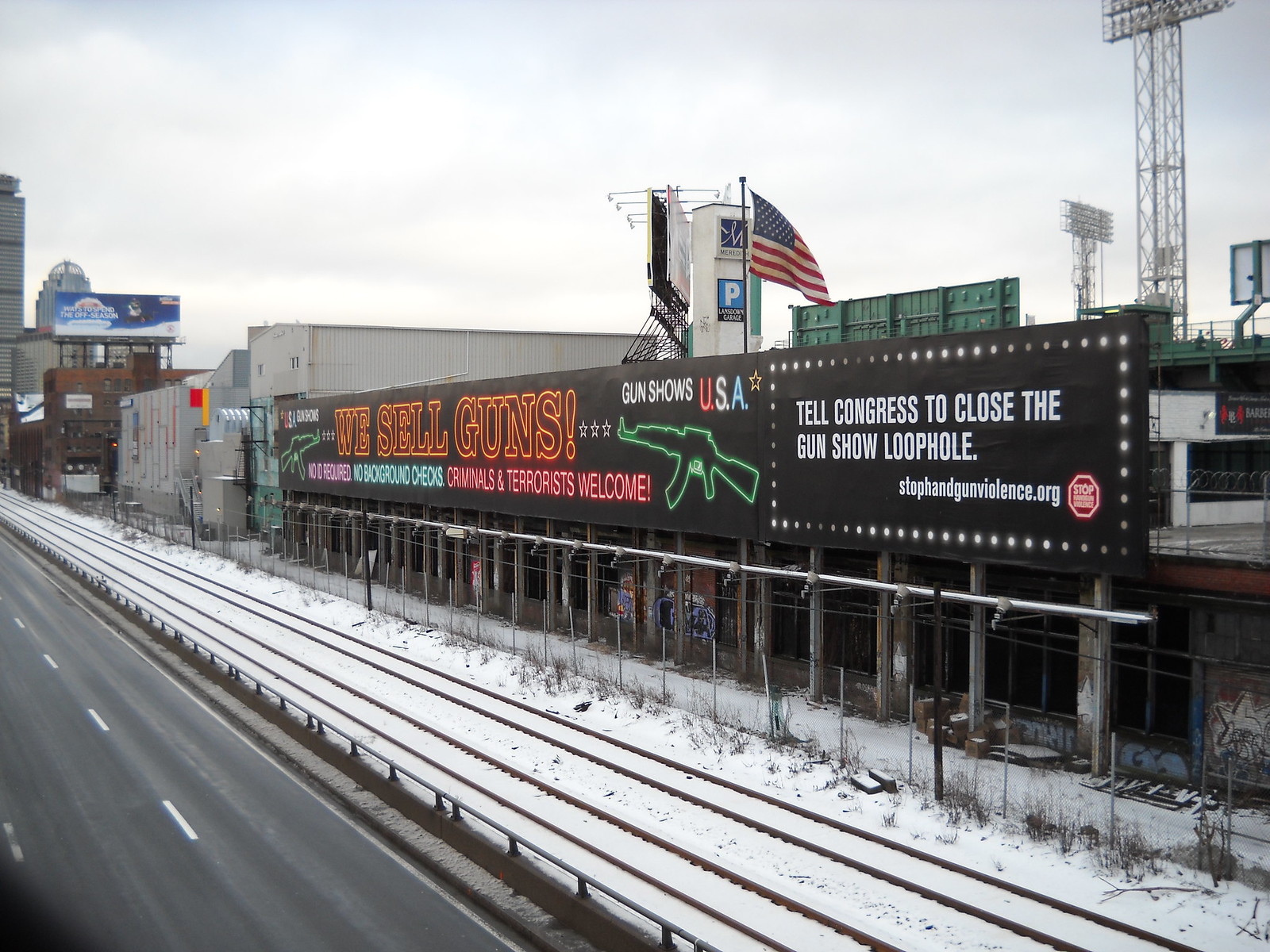This outdoor photograph captures a snowy urban scene on a cloudy day with a gray and white sky. The perspective is slightly elevated, looking down on a two-lane street on the left side, juxtaposed against a pair of snow-covered railroad tracks on the right. Beyond the tracks stands a series of buildings, including a dilapidated warehouse adorned with large, graffiti-tagged windows.

Dominating the image is a large, eye-catching billboard affixed to the warehouse. The billboard is brightly lit with green neon outlines of AR-15 style guns on both sides. Against a black background, the billboard prominently advertises "Gun Shows USA" at the top, with "We Sell Guns" in bold orange lettering in the center. Below this, the text reads "Delivered, No Background Checks, Criminals and Terrorists Welcome." Emphasizing the message, additional white text on the right side pleads, "Tell Congress to Close the Gun Show Loophole," promoting the website "StopHandgunViolence.org." An American flag is mounted above the billboard, waving in the somber atmosphere. The entire scene conveys a striking contrast between the chaotic urban elements and the serene, snow-covered surroundings.